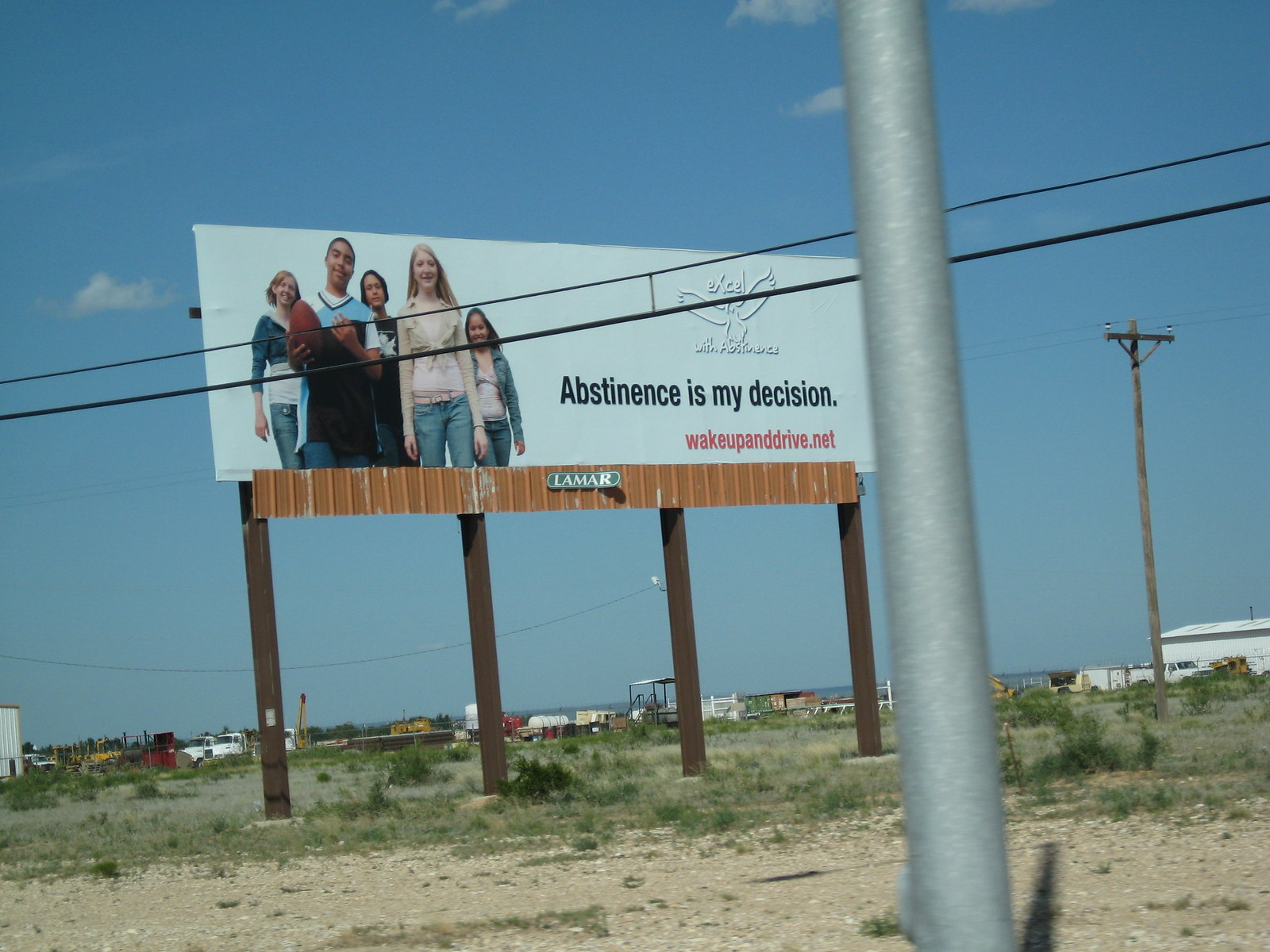In this daytime color photograph, a large white billboard stands tall on three robust steel I-beams, set against a background of clear blue skies with minimal clouds. The billboard's green oval logo prominently displays the company name, Lamar. Dominating the middle of the image, the billboard features a diverse group of five teenagers: three girls and two boys. Among them, two girls appear to be of European descent, one girl of African American descent, one boy is African American, and one girl may be Latina. The prominent message on the billboard reads in bold black text, "Abstinence is my decision," followed by a red website URL, wakeupanddrive.net. In the foreground, a large gray steel pole casts a shadow on the gravelly, weed-strewn ground, slightly obstructing the view. Utility wires cross the scene, and in the background, a distant telephone pole is visible along with a warehouse that houses a few trucks and some heavy yellow equipment, like a forklift.